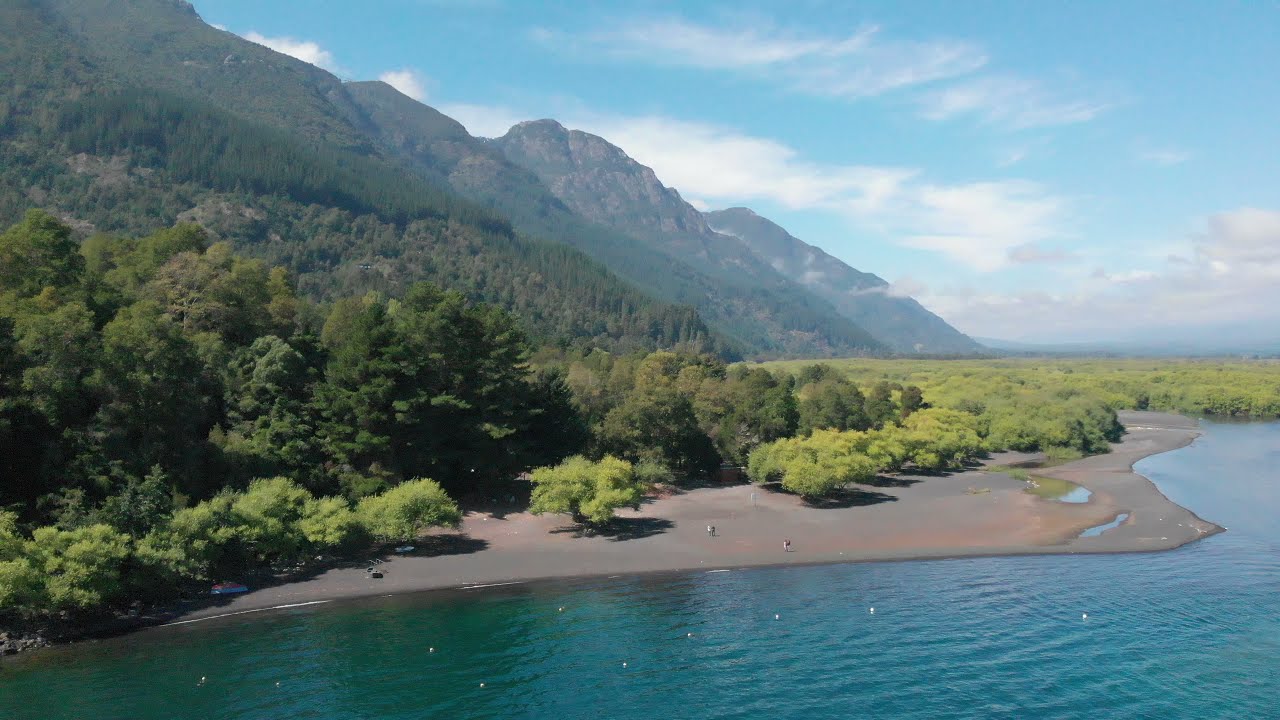The image captures an aerial view of an island surrounded by calm, blue-green water populated by several white birds, both in the water and on the rocky beach. In the foreground, the beach meets a flat expanse of short, light green trees, which are interspersed with sporadic greenery. Behind these, a line of larger, darker green trees, possibly pines, leads up to craggy, rocky mountains. These high mountains, marked by their rugged bluffs, dominate the center and left of the scene, with a bright blue sky filled with fluffy white clouds stretching above. On the beach, you can see a few people, a car parked under a tree, and buoys in the water for boats.